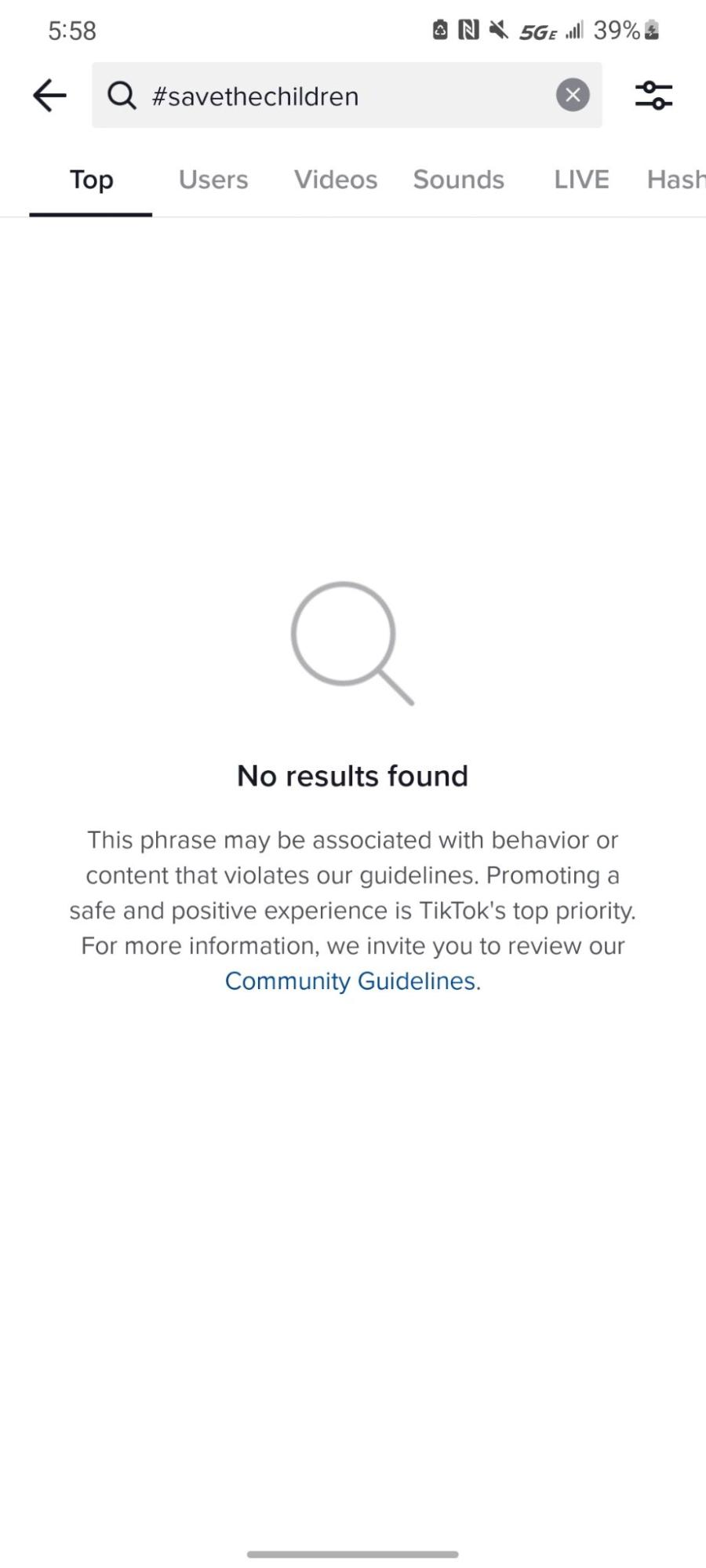This is a detailed screenshot of a TikTok search page. At the top of the image, the search bar contains the text "#savethechildren" in small grey font. To the left of the search box, there's a left-pointing arrow. Immediately below the search bar, there are several categories listed horizontally, with the "Top" category selected. 

The central part of the screen prominently features a large magnifying glass icon, accompanied by the message "No results found" in bold black font. Below this, a more detailed message reads, "This phrase may be associated with behavior or content that violates our guidelines. Promoting a safe and positive experience is TikTok's top priority. For more information, we invite you to review our Community Guidelines," with "Community Guidelines" in blue as a clickable hyperlink.

The background of the screenshot is white, maintaining a clean and simple interface. In the top-right corner, the status bar displays the battery icon, WiFi icon, and 5G icon. On the top-left corner, the time of the screenshot is visible. This image effectively captures TikTok's efforts to moderate content and ensure user safety by restricting search results for potentially harmful hashtags.